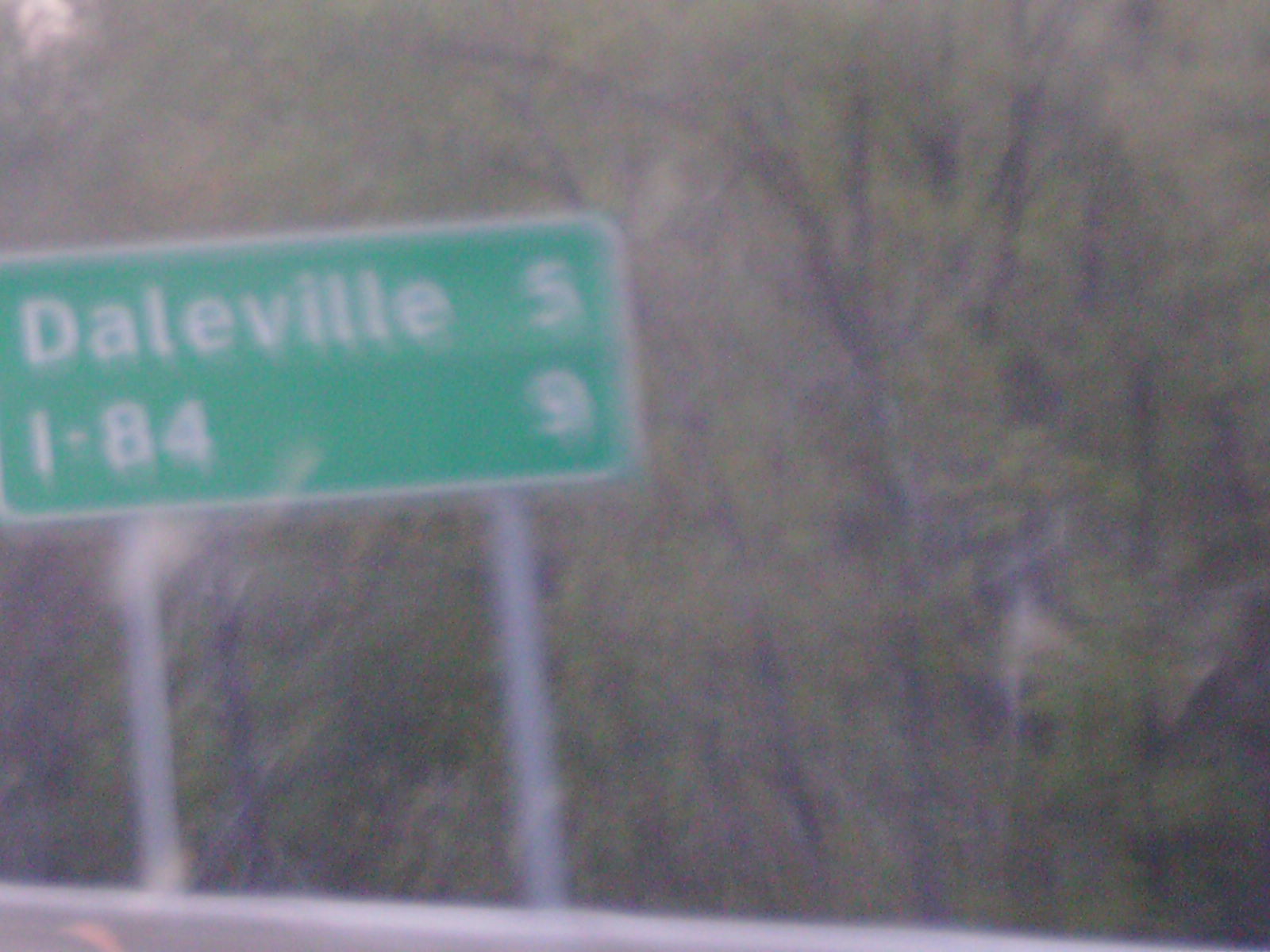The image captures a roadside scene, possibly taken while driving by a small town. A slightly blurry signpost, with a green background and white text, is featured prominently. The sign, which is mounted on wooden posts, reads "Daleville - 5 miles" and "I-84 - 9 miles." This sign is positioned amidst a collection of trees, some of which appear to be dead or barren, while others are lush with green leaves. A metallic guardrail runs along the left side of the scene. The vegetation surrounding the sign includes darker brown branches and green shrubbery. The photograph has a slightly aged appearance, with possible artifacts such as a small red speckle near the bottom left of the guardrail, suggesting it might be an old film photo that has been digitized.